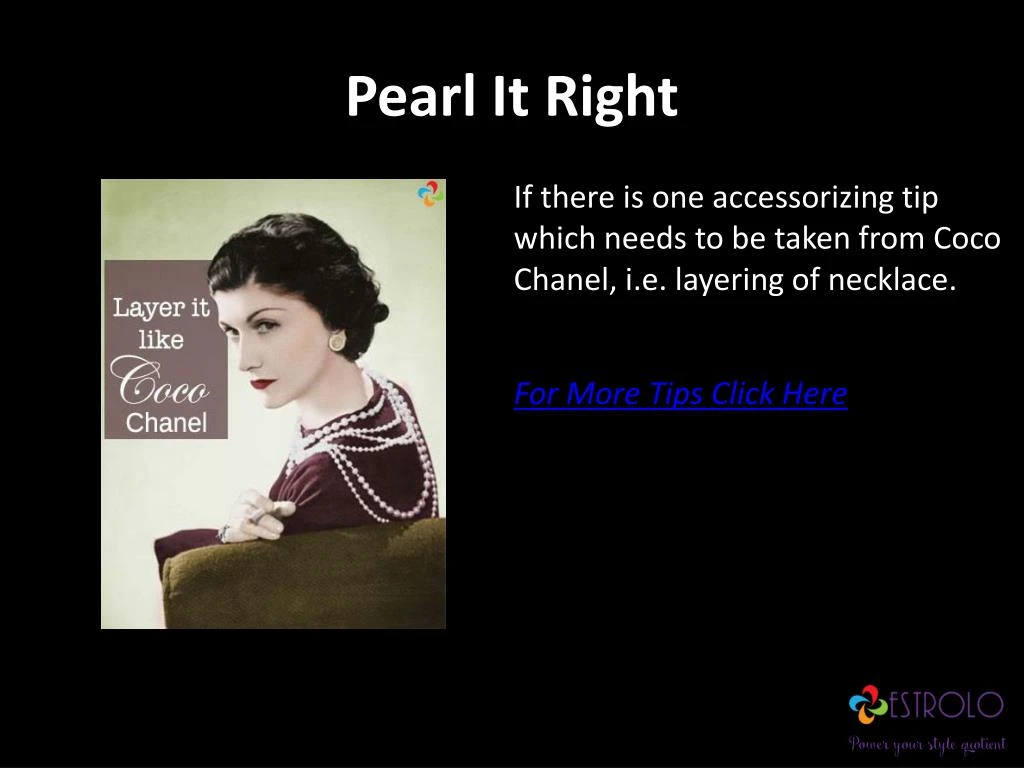The image features a black background with centered white text at the top reading "Pearl It Right." Beneath this, there is a rectangular, aged photograph on the left side. The photo, likely from the 1920s, showcases a woman with very light skin and dark, wavy bobbed hair. She has dark red lips and is dressed in a dark top with a gloved hand holding a cigarette. Multiple strings of pearls drape elegantly over her shoulders and back. The background of the photograph appears light-colored, possibly greenish, and there is a text overlay on the photo saying "Layer It Like Coco Chanel." To the right of the photograph, still on the black background, more white text reads, "If there is one accessorizing tip which needs to be taken from Coco Chanel, i.e. layering of necklaces." Below this, blue underlined text invites the viewer to "For more tips, click here." In the bottom right corner, there is a subtle logo in light lettering for "Estrolo."